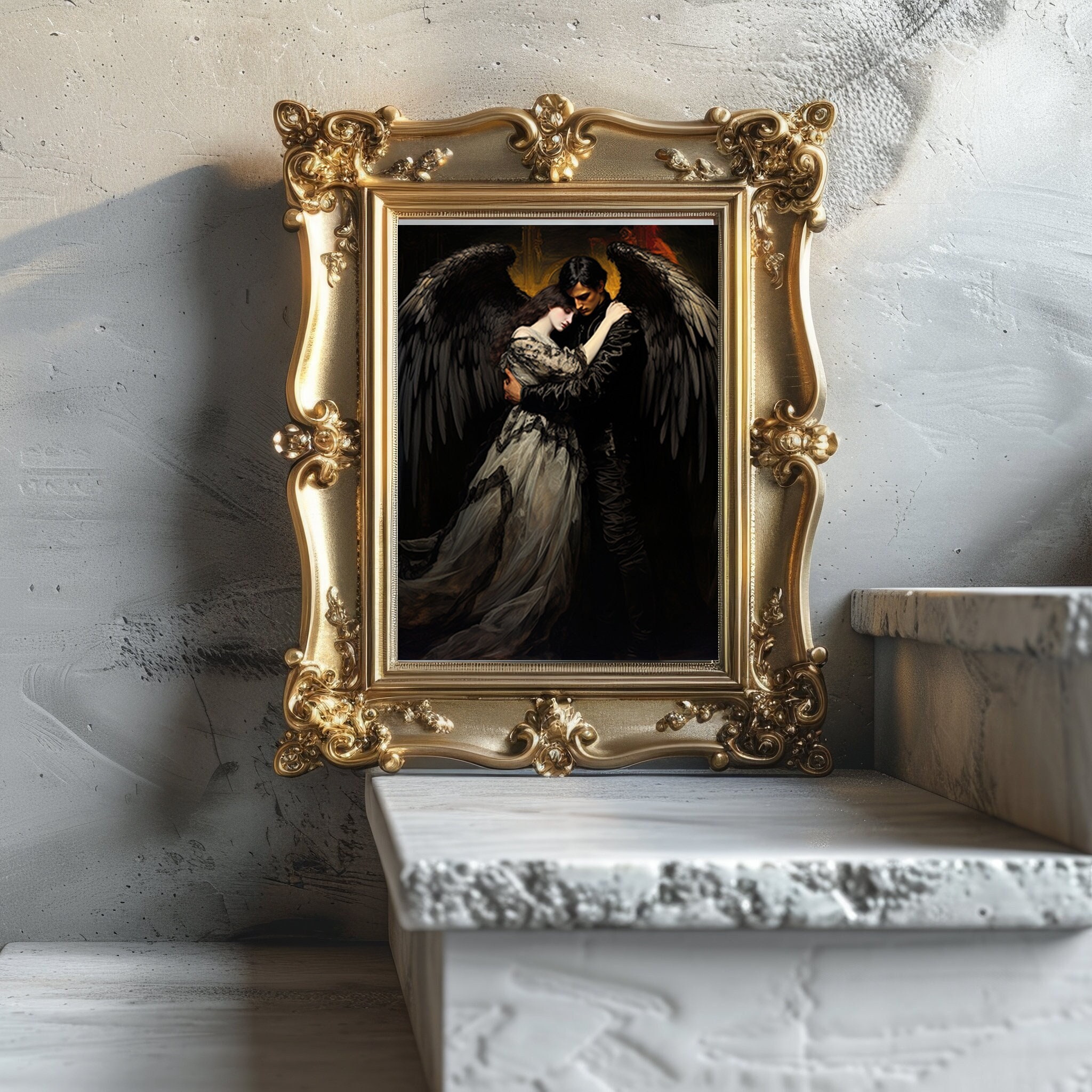This image showcases a detailed scene of a high-end, fantasy-themed painting in an ornate golden frame, resting on the first step of a light gray, stone staircase. The painting, framed elaborately with decorative accents at the corners and midsections, features a man and a woman with sorrowful expressions embracing each other. The man, dressed in an old-fashioned black suit, has large, majestic black wings sprouting from his back, framing the upper corners of the image. The woman, holding onto him, is depicted with pale skin and long brown hair, wearing a Victorian-style gown of gray and black. The trio is placed against a light gray, plaster wall with intricate etchings, creating a sophisticated and slightly distressed backdrop.